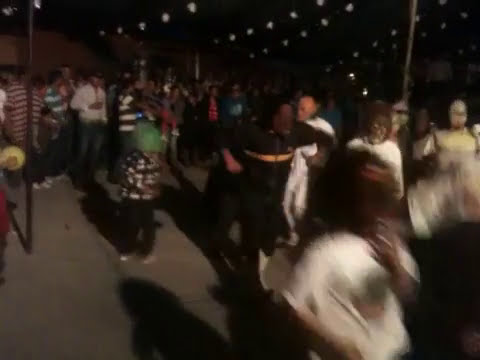The image depicts a lively nighttime gathering with numerous people on what appears to be a gray cement floor, potentially an outdoor setting. The ambiance is dim, illuminated by rows of string lights, reminiscent of Christmas lights, hanging above the scene. Among the crowd, several individuals are holding drinks. The scene is somewhat chaotic; some people near the forefront seem to be dancing, while others in the background appear stationary. Despite the overall blurriness and poor quality of the photo, which obscures detailed facial features and makes discerning specific activities challenging, the festive atmosphere is palpable. A few attendees are dressed in costumes or masks, suggesting a possible Halloween theme. The predominant attire visible includes white shirts and various striped shirts in blue, gray, red, and white hues. Overall, the image captures a bustling and spirited event, albeit with indistinct and hazy visuals.